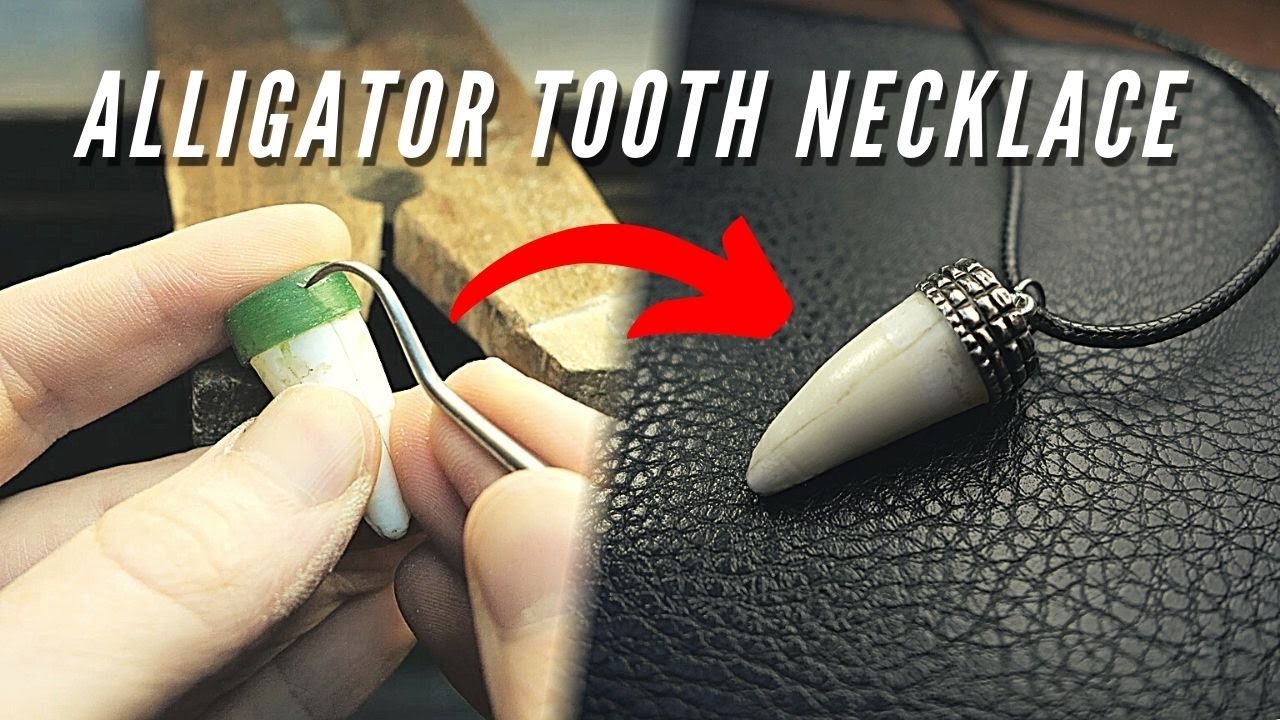The image depicts the detailed creation of an alligator tooth necklace. At the top, bold italicized white text prominently displays "alligator tooth necklace." Centrally, two light-skinned hands are actively working on the tooth; the left side shows one hand holding the white alligator tooth, which features a green cap. The other hand maneuvers a shiny silver pick, piercing into the green cap. A prominent red arrow points towards the tooth, highlighting it.

In the background, there's an object resembling a giant wooden clothespin, providing a subtle backdrop to the meticulous crafting process. The right side of the image showcases the finished necklace, resting on a black leather surface. The tooth is capped with silver, designed with rectangular scales, and attached to a black, somewhat shiny cord. The tooth's top part appears slightly cracked, adding a touch of authenticity to the crafted piece.